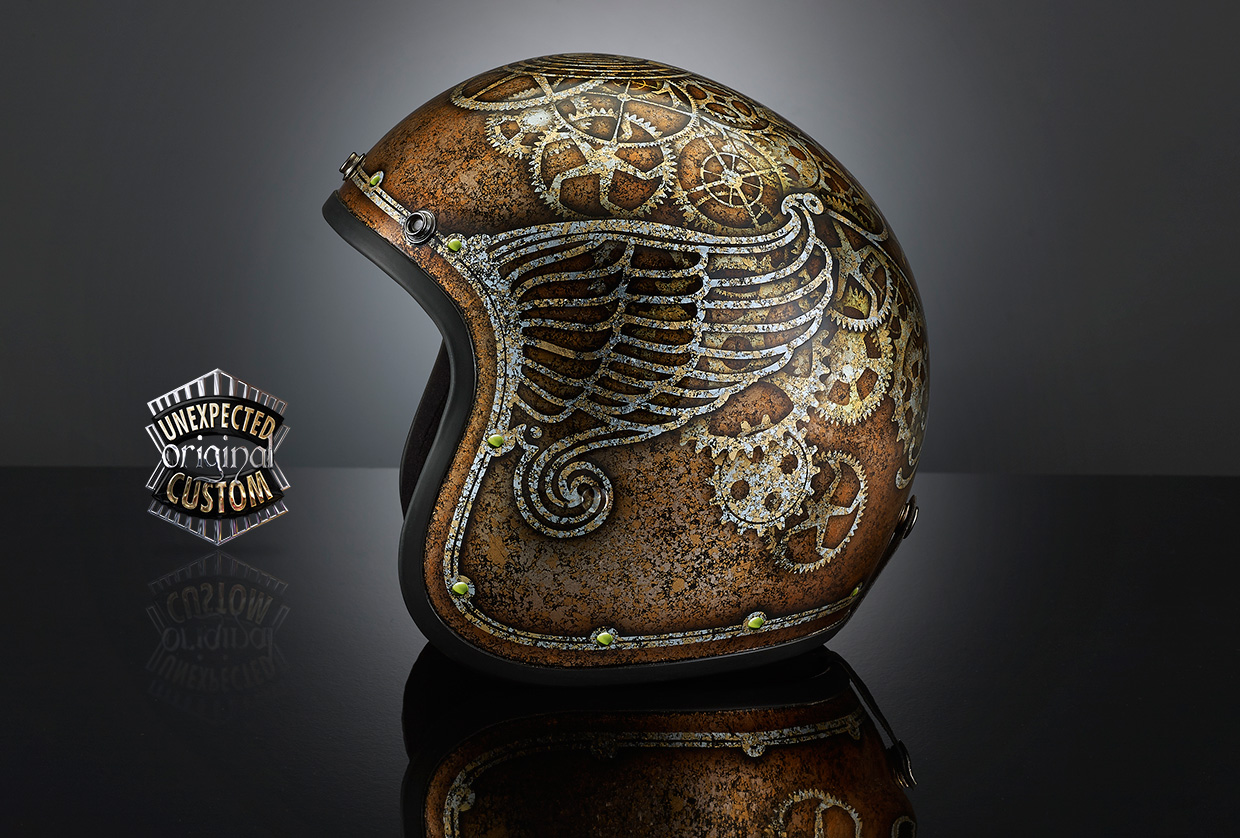The image showcases a meticulously detailed, custom-painted helmet positioned on a reflective black surface, with a dark gray background that accentuates its features. The helmet, facing left, is predominantly crafted in a dark brown hue adorned with black speckles, and features intricate dark gold and bronze trim all around its edge. Prominent black and double gray lines frame the helmet, adding depth to its design.

Notably, the helmet is embellished with metallic, steampunk-inspired gears and cogwheels of varying sizes and shapes, each rendered with little vertical lines representing teeth, and extending from the top to the back of the helmet. On the sides, finely detailed gold and silver wings with feathers—exuding a swirly, fluid design—add to its visual appeal. Additionally, small green jewels are subtly placed on the left side, offering a touch of vibrant contrast.

In the foreground, the text "Unexpected Original Custom" is positioned next to the helmet alongside a logo, reinforcing the uniqueness of the piece. The overall setting and professional photograph highlight the helmet's craftsmanship and artistic elements.